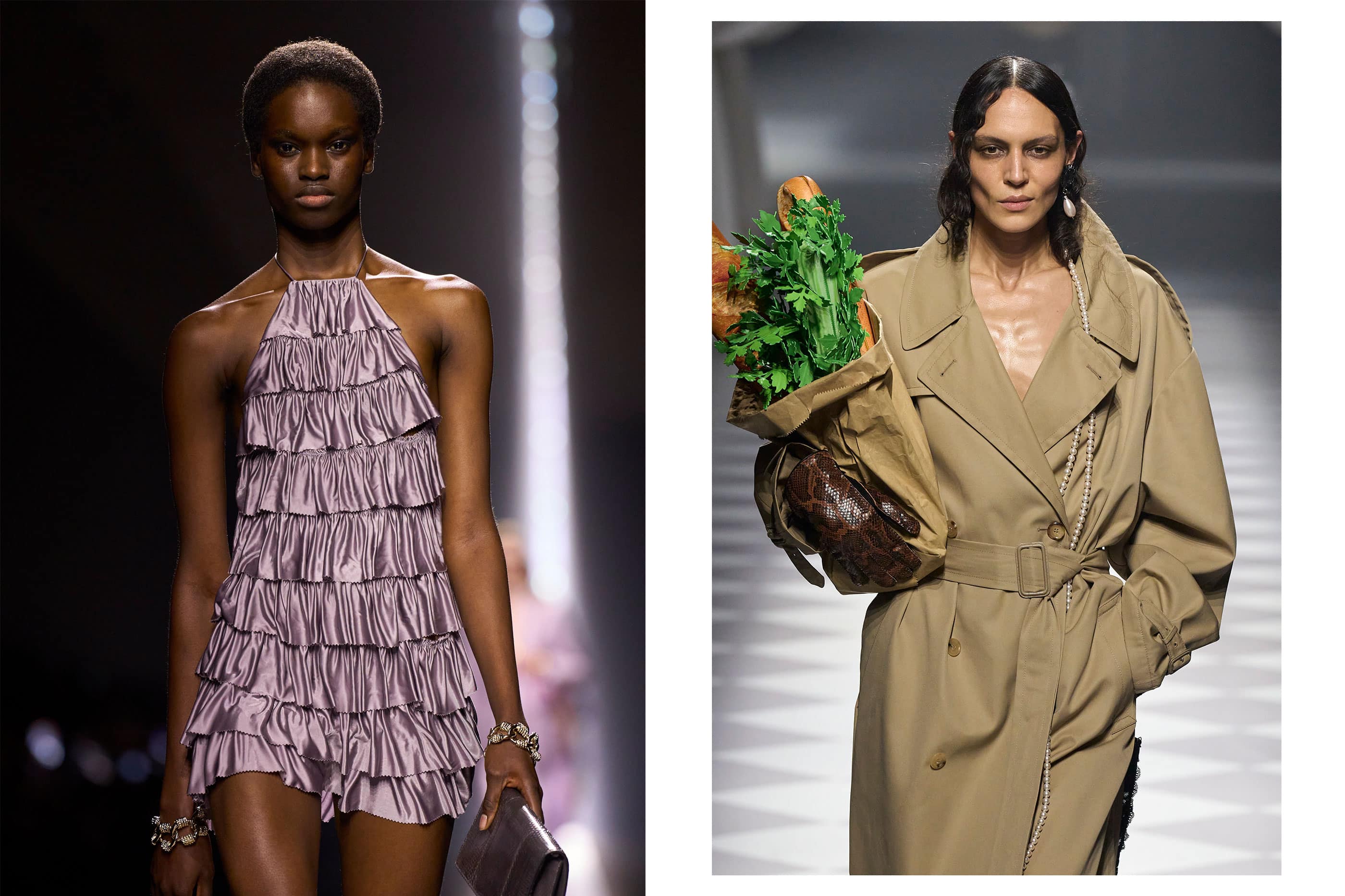This image features two side-by-side color photographs of runway models. On the left, an African American woman with very short black hair is staring forward with a serious expression. She dons a light purple, shiny satin outfit that features ruffled details and a halter-style neckline, exposing her shoulders and arms. Her ensemble is complemented by silver bracelets on both wrists, and she carries a black purse in her left hand. The background behind her is black, highlighting her striking appearance.

On the right, another model with long, dark hair, possibly of Hispanic or South American descent, walks on a black and white checkerboard floor. She is wearing a beige trench coat, seemingly with nothing underneath, cinched at the waist with a matching belt. Around her neck is a long pearl necklace that extends below her waist. In her arms, she carries a brown paper bag filled with greenery and a French baguette. Her expression is one of subtle amusement, adding a playful contrast to the scene.